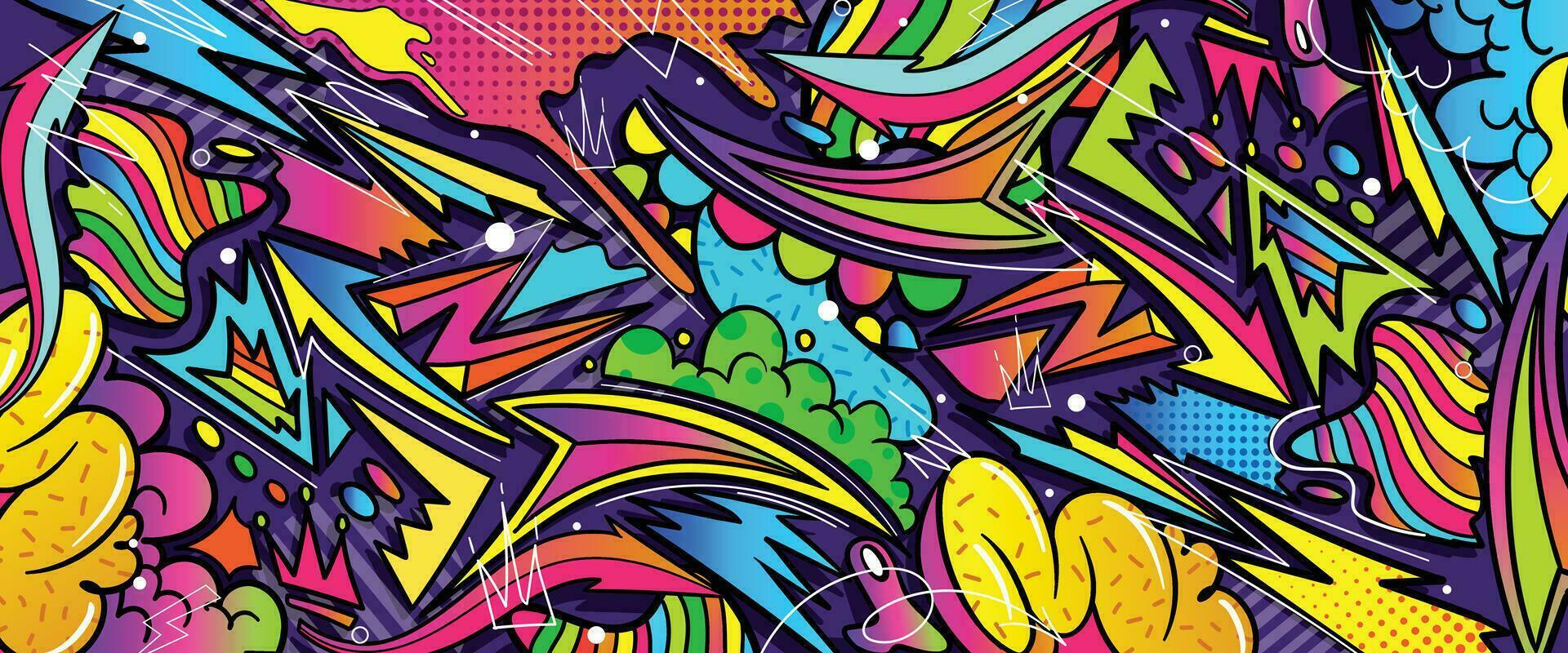This vibrant artwork resembles a mix between abstract graffiti and vector art from the 1970s, with an explosion of colors spanning red, orange, green, blue, pink, yellow, turquoise, and dark green. The design features a chaotic blend of solid-colored shapes, gradient fill patterns, and black outlines, creating an energetic and dynamic composition. Throughout the piece, you can find multicolored stripes in combinations like yellow and red, blue and red, semi-circles in colors like blue, yellow, and red, and green cloud-like forms. Additionally, the artwork includes various random and organic doodles, such as half-tone patterns, and prominent arrows and small crowns drawn in white over the vivid background. The imagery lacks uniformity and recognizable forms, giving it an informal, doodle-like quality typical of street art.